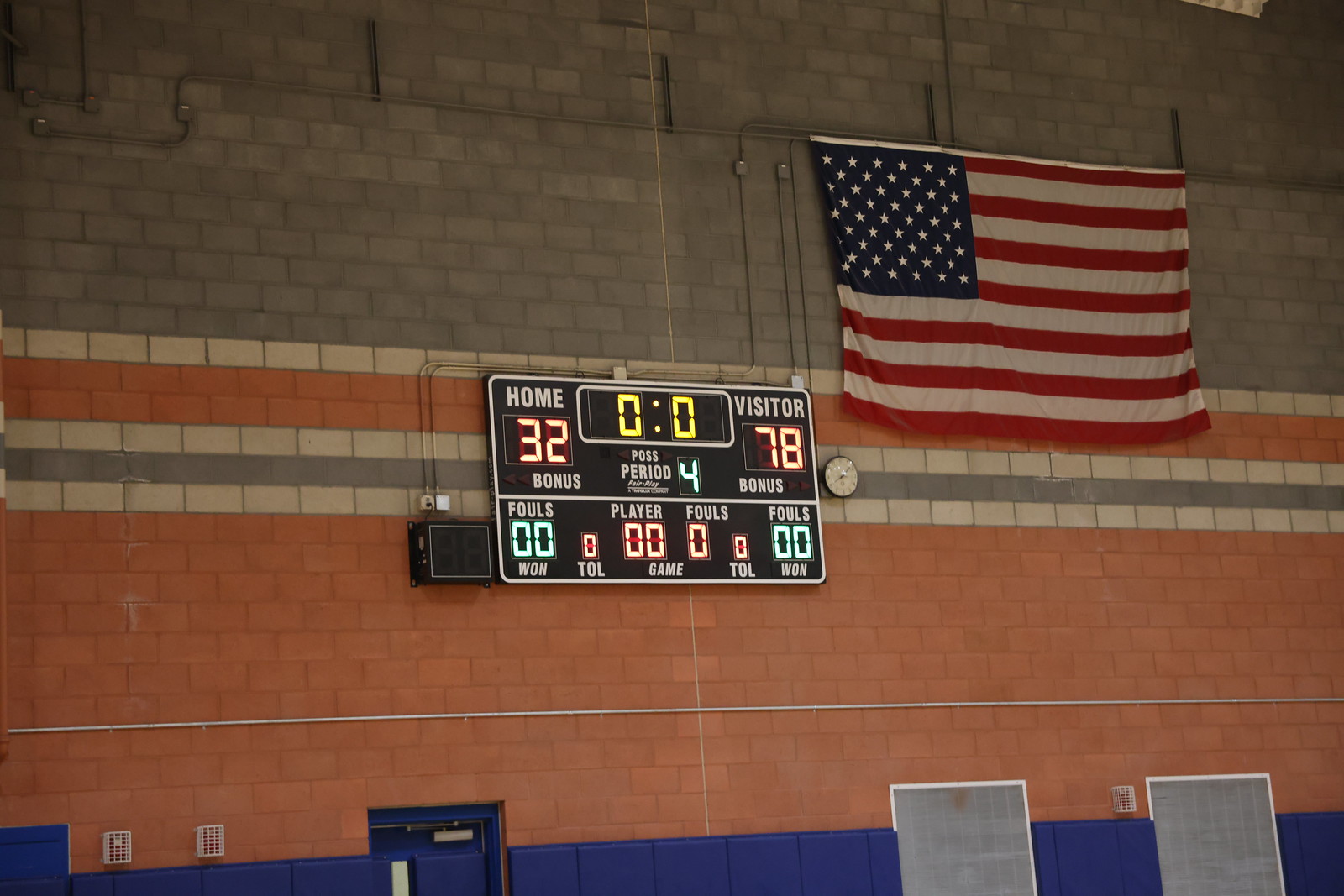This photograph captures the interior of a high school gymnasium. Prominently featured is a multi-colored cinder block wall, with a dark grey top that transitions through stripes of white, grey, and orange brick, down to dark blue padding along the bottom, near several door frames. Central to the image is a black scoreboard indicating a final score of 32-78 in favor of the visiting team, with the time expired in the fourth period. Adjacent to the scoreboard, slightly higher and to the right, an American flag drapes against the wall, its red and white stripes and blue field of stars clearly visible. To the left of the scoreboard, a small clock is mounted. The overall impression is one of a typical yet detailed high school gym setting, complete with the customary elements of padding, scoreboards, and patriotic decor.